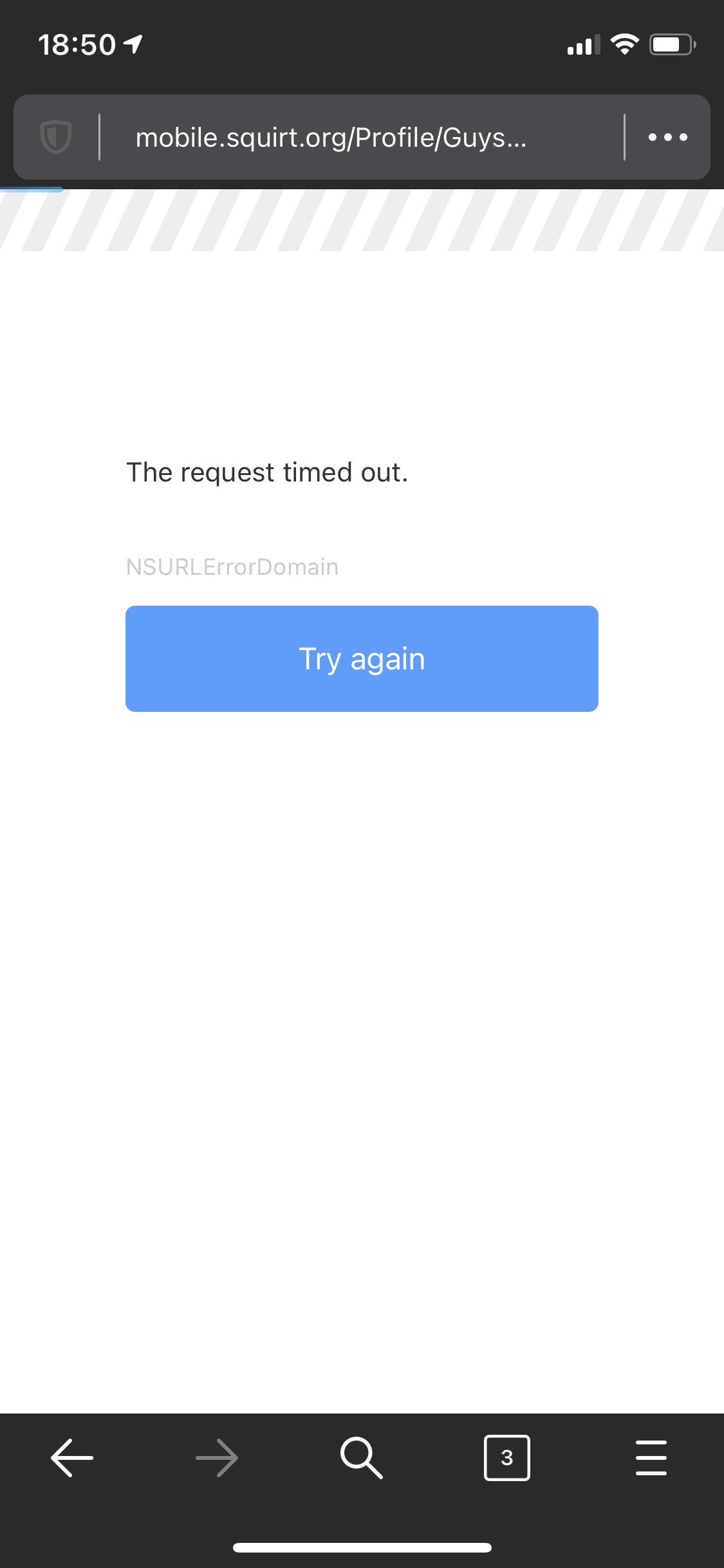A screenshot from a mobile app displays an error message indicating that the request has timed out. The upper portion of the screen features a black search bar with the text "mobile.squirt.org Profile Guides". Directly below this, a prominent error message reads, "The request has timed out," accompanied by a blue "Try Again" button. At the bottom of the screen, a black navigation bar includes several icons: a back arrow, a forward arrow, a zoom icon, a square icon with the number three, and a set of three horizontal lines, whose function is unclear. This image clearly shows a network or server issue encountered while attempting to load a specific profile guide on the app.